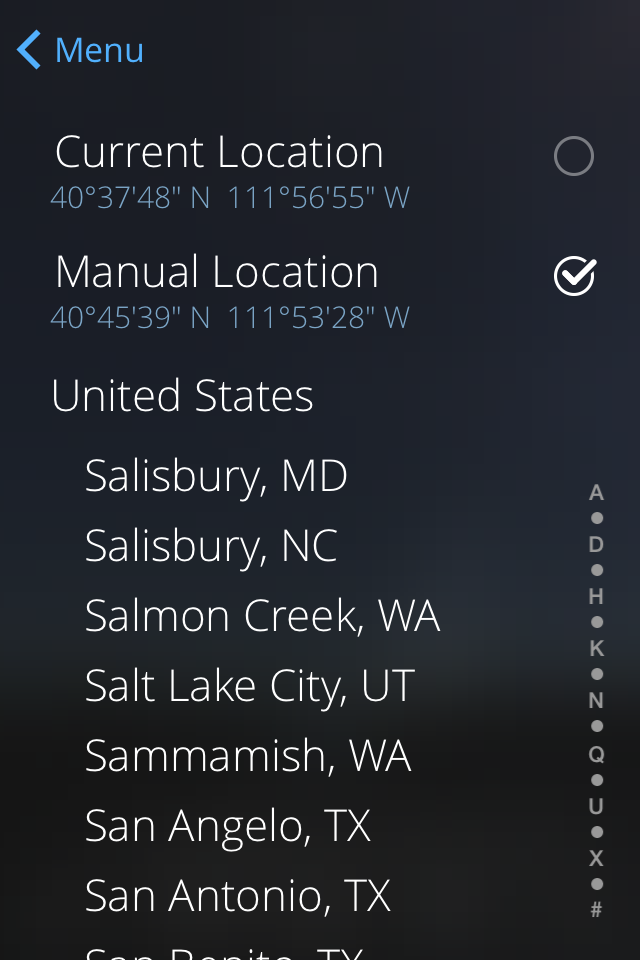The image depicts a black rectangular interface. In the upper left-hand corner, there is an arrow pointing to the left labeled "Menu." Below this, the text "Current Location" appears in white. Underneath, in blue text, the geographical coordinates are displayed as "40° 37' 48" N, 111° 56' 55" W." Next to these coordinates is a grey outlined circle with the text "Manual Location" in white.

To the right of this circle is another circle containing a check mark, followed by another blue text displaying additional coordinates for north and west directions. Below these elements, the names of various locations in the United States are listed: Salisbury, MD; Salisbury, NC; Salmon Creek, WA; Salt Lake City, UT; Samamish, WA; San Angelo, TX; and San Antonio, TX.

On the right side of the interface, letters of the alphabet are displayed, each followed by a grey circle: A (with a dot underneath), D (with a grey circle underneath), H (grey circle), K (grey circle), N (grey circle), Q (grey circle), U (grey circle), X (grey circle), and a hashtag symbol (#).

This detailed interface layout presumably allows the user to select or manually enter a location, with a focus on geographical coordinates and a list of selectable areas.